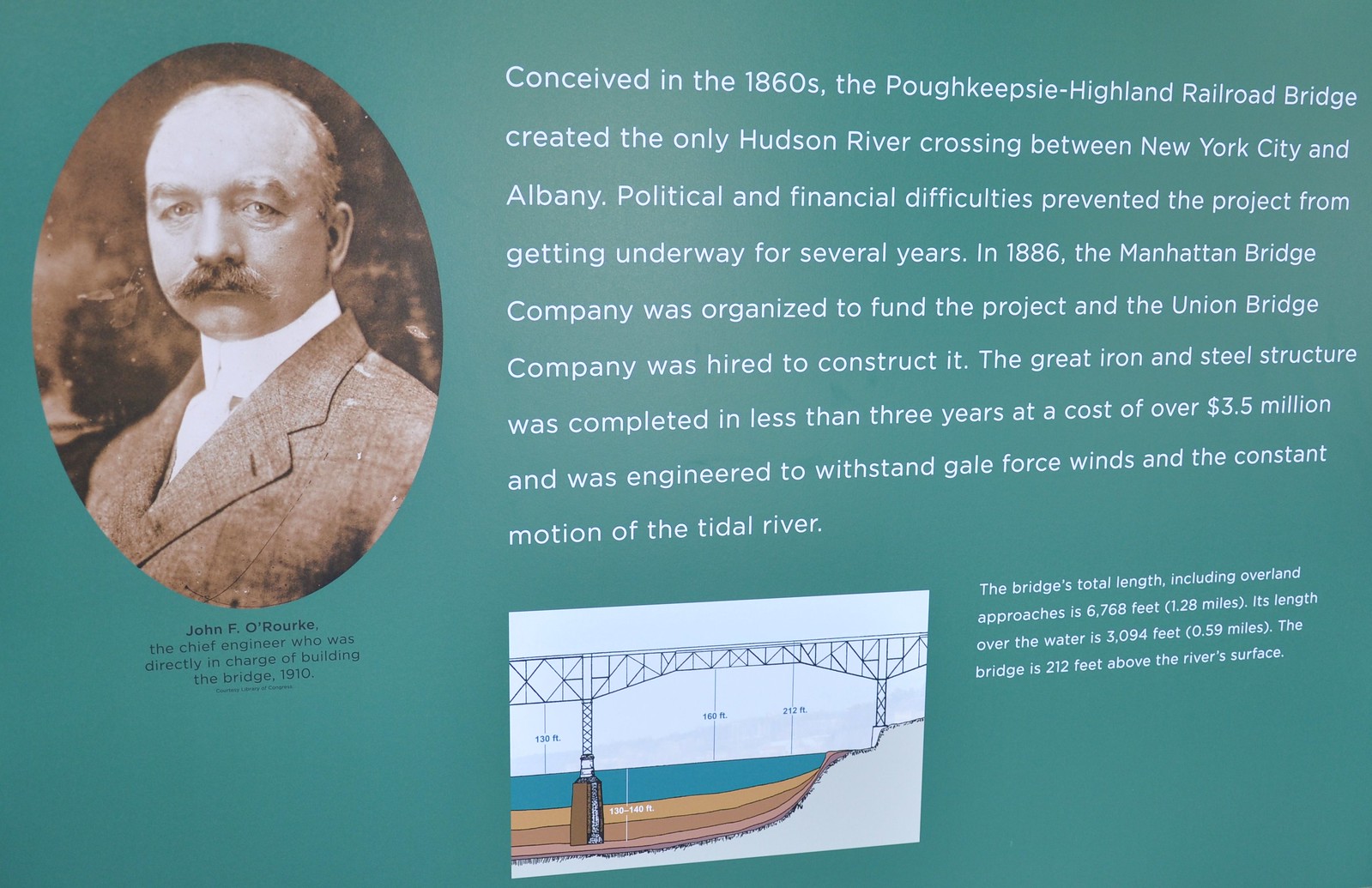A museum-style sign with a teal green background features an oval sepia-toned photograph of an older man with a receding hairline, bushy mustache, and light-colored eyes, dressed in a high-collared white shirt and suit jacket. The caption beneath the photograph identifies him as John F. O'Rourke, the chief engineer who was directly in charge of building the Poughkeepsie Highland Railroad Bridge in 1910. Next to the photograph, white text on the green background details the bridge's history: "Conceived in the 1860s, the Poughkeepsie Highland Railroad Bridge created the only Hudson River crossing between New York City and Albany. Political and financial difficulties delayed the project for several years. In 1886, the Manhattan Bridge Company was organized to fund the project, and the Union Bridge Company was hired to construct it. The great iron and steel structure was completed in less than three years at a cost of over $3.5 million and was engineered to withstand gale force winds and the constant motion of a tidal river." Below this text is a black-and-white line drawing of the bridge, showing the river underneath and the depth at which the bridge's pilings are driven into the riverbed. The sign further informs that "The bridge's total length, including overland approaches, is 6,768 feet (1.28 miles). Its length over the water is 3,094 feet (0.59 miles). The bridge is 212 feet above the river's surface."